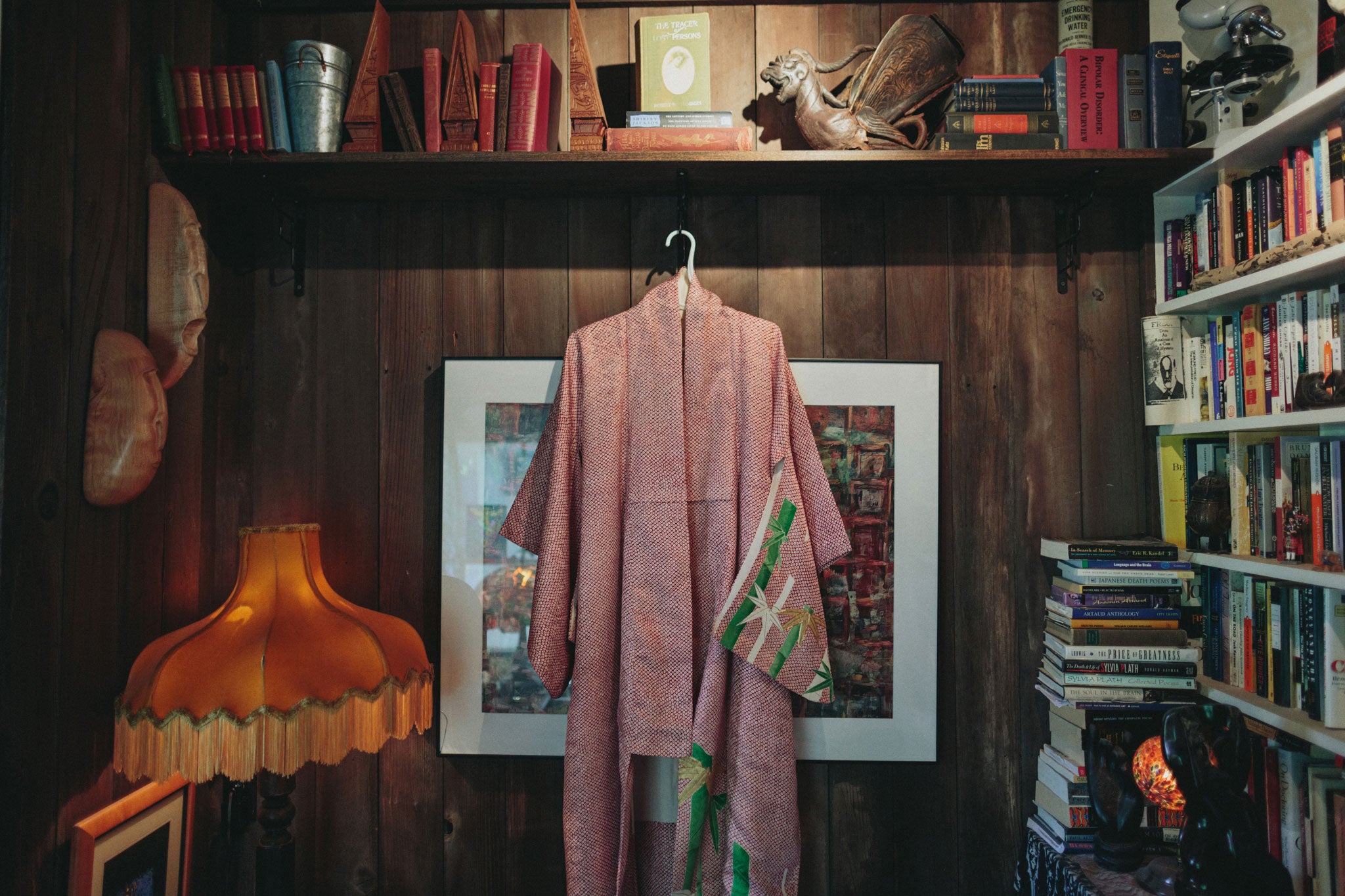The image depicts a cozy reading nook or a small enclosed room with wood-paneling. On the right side, there is a white bookshelf completely filled with books, showcasing the occupant's love for reading. In front of the bookshelf, a small table is piled with additional books. The focal point of the image is a pink and white kimono, adorned with decorative green and white leaves, hanging from a white hanger on a hook. This kimono partly obscures a framed painting on the wall behind it. Above the kimono, a shelf brims with more books and various knickknacks, including some figurines. The left side of the image features a fringed, chandelier-like table lamp with an orange shade, probably a vintage piece from the 70s. Additional knickknacks adorn the left wall, where another picture is also displayed. This space might serve as a reading nook or simply an area for book storage.